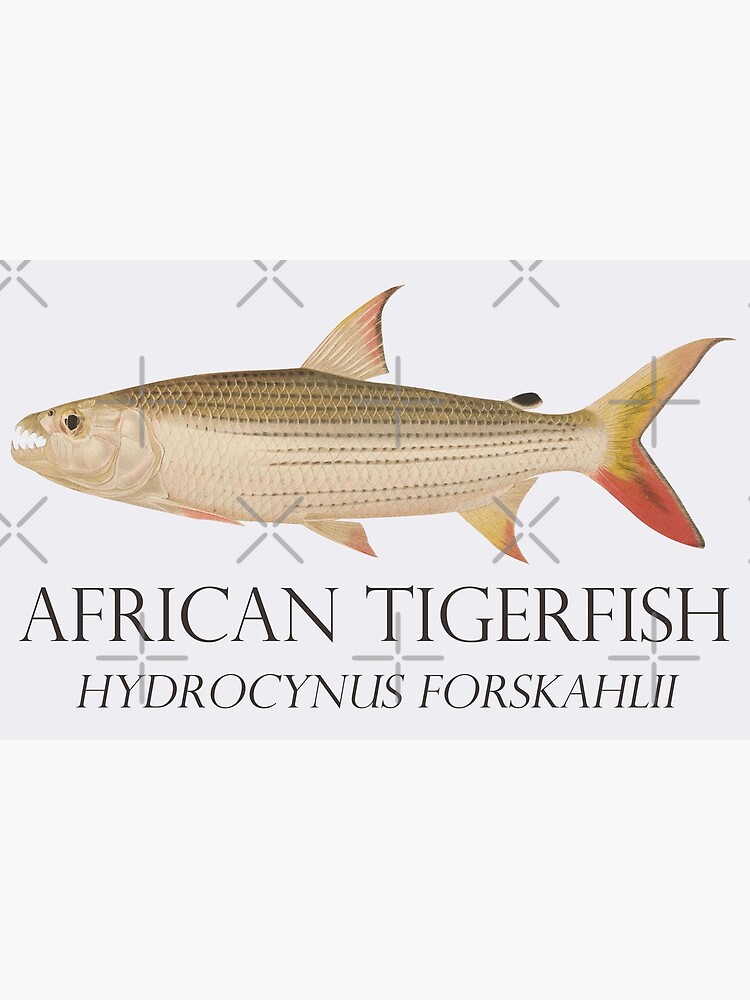The poster illustration features a beige African tiger fish, distinguished by its sharp, prominent teeth and menacing appearance. The fish's coloration includes a darker brownish top, with reddish-orange and yellow highlights on the tail and fins. Its large, alarmed dark brown eye is also prominent. Below the fish, in bold uppercase black text, the name "African Tiger Fish" appears, followed by the scientific name "Hydrocynus forskallii" in slightly less bold but still uppercase letters. The background consists of a light gray backdrop with a darker gray rectangle where the fish is placed. The entire image is overlaid with a watermark of gray crosshatches, likely to prevent unauthorized use.